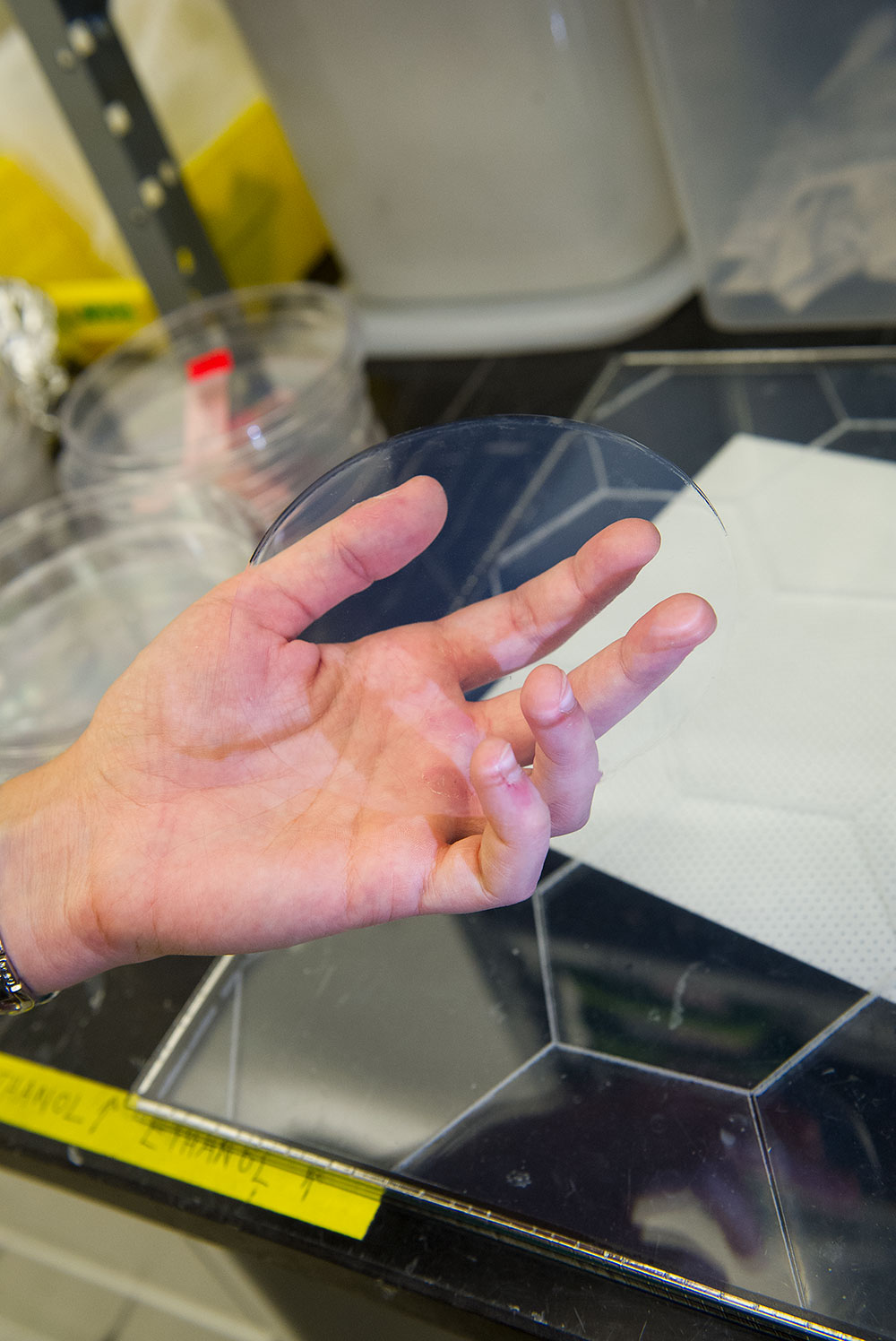The photograph depicts a close-up view of a person's left hand gently holding a semi-transparent, light-colored circular object, possibly a glass Petri dish, with their palm facing upwards and fingers lightly pressing against it. The person, whose skin tone appears to be Caucasian, wears a silver metal wristwatch on their wrist. The photograph is rectangular, with its longer sides on the left and right, and is taken indoors. The background features a black countertop with a distinct hexagonal tile pattern. Resting on the countertop is a square-shaped glass board, atop which lies a piece of paper towel. To the left of the hand, there are multiple sample discs or glass Petri dishes, while the top right of the image displays stacked plastic storage containers. Positioned on the countertop is a yellow sticker labeled "ethanol." The setting, characterized by these elements, suggests a laboratory environment.